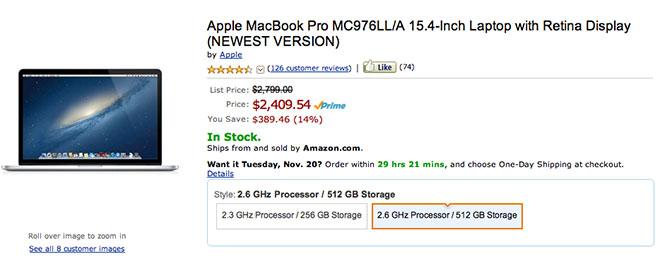This image showcases an Amazon product page for an Apple MacBook. On the left side of the screenshot, there's a picture of the MacBook, prominently displaying a blue screen and the sleek silver edges of the keyboard. The right side contains detailed product information in black text. The product is described as an "Apple MacBook Pro MC976LL-A 15.4-inch laptop with Retina display," and is noted as the newest version. The listing shows a rating of 4.25 stars based on 126 customer reviews.

Beneath the product name, there is a line separating the details. The original list price of $2,799 is crossed out, highlighting a discounted price of $2,409.54 in red, accompanied by a checkmark and Amazon Prime logo. An additional note informs that the discount saves the buyer $389.46, which is a 14% reduction from the original price. Finally, the availability is indicated in green letters: "In stock, ships and sold by Amazon.com."